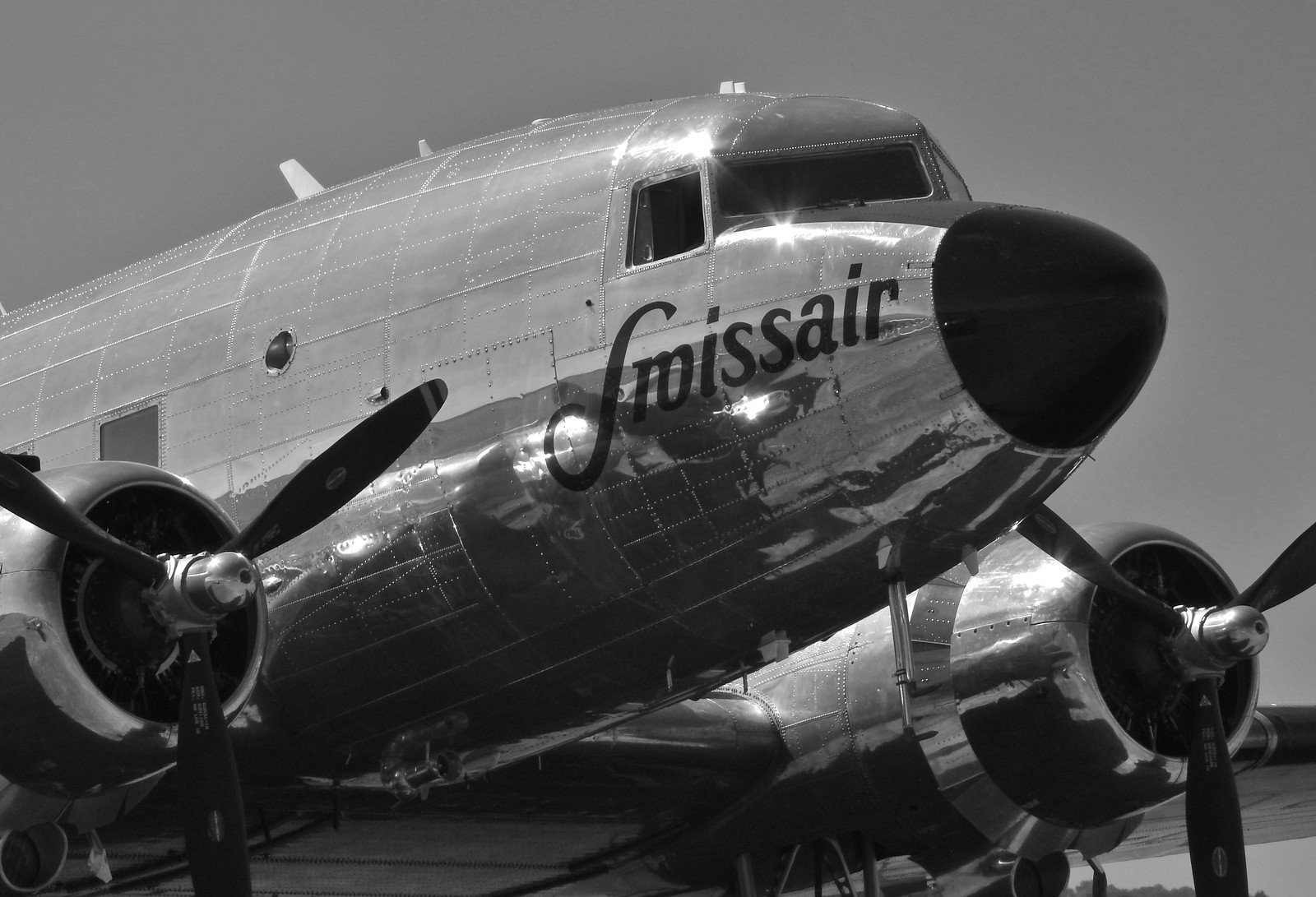This black and white photograph showcases a large, old-style, silver propeller airplane with a shiny, reflective surface. Prominently, the aircraft features a big black nose, which almost resembles the face of a dog upon closer inspection. The plane has two propellers on each side. There are small windows in the cockpit, with one window open in the middle of the image. The black lettering on the side of the aircraft spells out either "L-M-I-S-S-A-I-R" or "S-I-O-I-S-S-A-I-R" in a slightly fancy script. The concrete tarmac and a gray sky serve as a backdrop, adding to the vintage atmosphere of the scene.